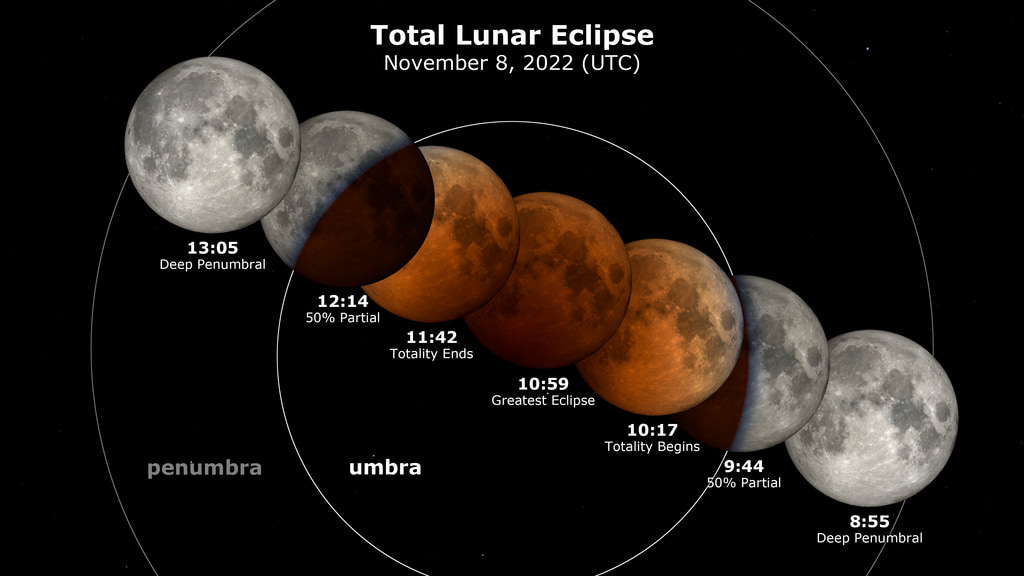This image is a detailed diagram of the total lunar eclipse that occurred on November 8th, 2022, in UTC. Titled "Total Lunar Eclipse" in white text at the top, the diagram maps out the eclipse's various stages with time stamps, illustrating the moon's journey through the Earth's penumbra and umbra. 

The graphic features concentric circles: the inner circle represents the umbra (the fully shaded inner region), and the outer circle depicts the penumbra (the partially shaded outer region). Within these circles, seven distinct phases of the moon during the eclipse are displayed in a sequence starting from the top left and proceeding to the bottom right.

The stages and their corresponding times are as follows:
- 13:05 (Deep Penumbral)
- 12:14 (50% Partial)
- 11:42 (Totality Ends)
- 10:59 (Greatest Eclipse)
- 10:17 (Totality Begins)
- 09:44 (50% Partial)
- 08:55 (Deep Penumbral)

The image appears to use real photographs of the moon arranged in a visual diagram, showing the moon's progression through the penumbral and umbral shadows. The only colors in the image are the grey shades of the moon in the penumbral stages and the red hues when the moon is fully in the umbra, emphasizing the visual phases of the eclipse.